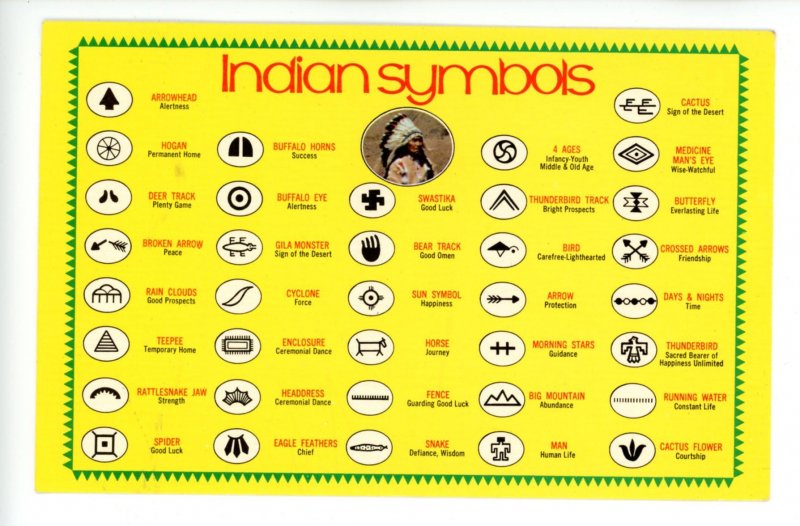This scanned image showcases a yellow chart with a green triangular patterned border, detailing Native American symbols and their meanings. At the top, in bold red letters, it reads "Indian symbols." The chart is organized in five columns, each displaying various symbols in black within white circles. In the center, there's an illustration of a Native American adorned in a feathered headdress.

The chart includes descriptions of each symbol alongside their associated meanings. For instance, an arrow is labeled "Arrowhead" and signifies alertness, while a wagon wheel-like symbol is described as "Hogan" representing a permanent home. Other symbols include a broken arrow meaning peace, a spider symbolizing good luck, and a deer track representing plenty of game. Additional symbols such as Rain Clouds for good prospects, Teepee for a temporary home, Rattlesnake Jaw for strength, Buffalo Horns, and a bullseye called Buffalo Eye are also depicted. Overall, the chart presents approximately thirty of these black-and-white emblems with detailed explanations in red print.